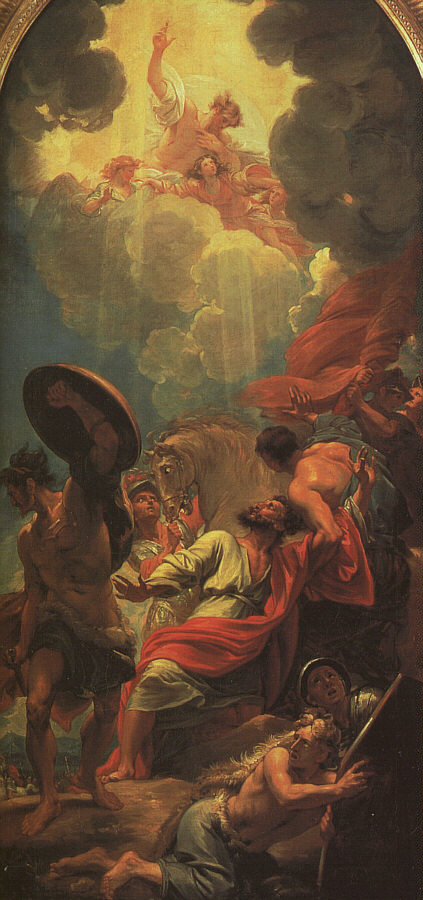This captivating Renaissance-style religious painting is teeming with intricate details and emotional storytelling. At the bottom, a half-naked man in blue pants lies on the ground, looking upwards, accompanied by another man whose head alone is visible. In the center, the scene appears tumultuous, reminiscent of a battle or abduction, with several men clad in robes. One of these central figures, a dark-haired and bearded man in a white robe with a red sash, is collapsing backward, seemingly fainting, while another man attempts to hold him up. Beside them, a muscular warrior grips a bronze shield and another man holds the reins of a light brown horse. Above, the sky is a dramatic tapestry of dark gray clouds, some with almost human-like faces, giving way to fluffier white clouds and rays of sunlight beaming down. At the zenith of this celestial gathering are angels – three female angels dressed in pink, and one larger male angel with red hair and no shirt, all floating ethereally among the clouds with their arms outstretched, seeming to oversee the chaotic events below. This masterpiece seamlessly blends the divine with the terrestrial, capturing a timeless struggle infused with spiritual poignancy.